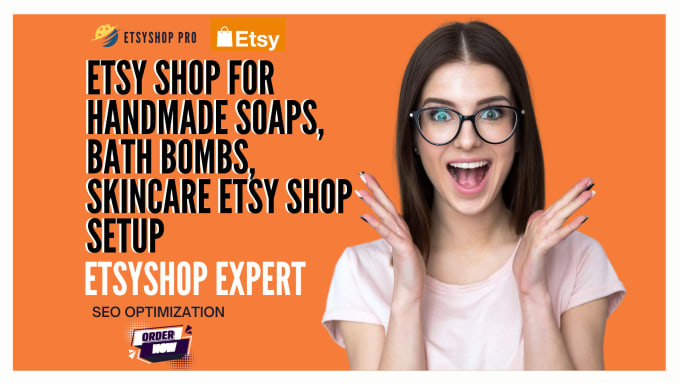The promotional image for an Etsy shop features a vibrant orange background with prominent black and white text. At the top left corner, a globe icon labeled "Etsy Shop Pro" is followed by a white shopping bag icon labeled "Etsy." The central text in the image reads, "Etsy Shop for Handmade Soaps, Bath Bombs, Skincare, Etsy Shop Setup, Etsy Shop Expert, SEO Optimization," and concludes with a call to action, "Order Now," in varying block lettering. To the right, a woman with shoulder-length brown hair, wearing black glasses and a light pink top, displays an enthusiastic, wide-open mouth smile with her hands raised and fingers spread, capturing her excitement.